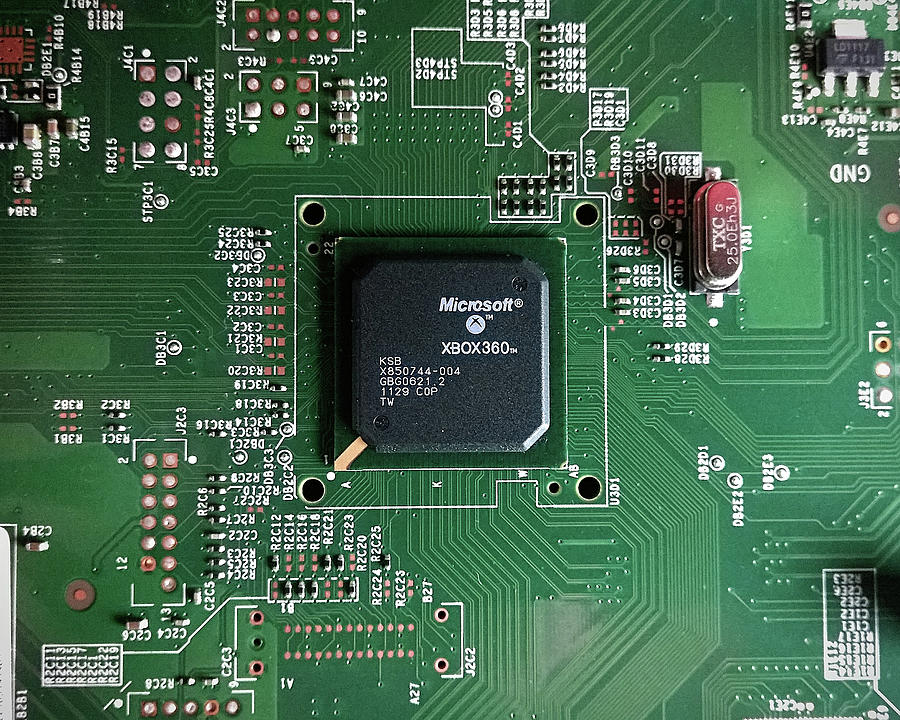The image showcases the intricate interior of a Microsoft Xbox 360 console, specifically focusing on its motherboard. The entire background is a sprawling, organized expanse of green, dotted with lighter and darker shades. Tiny, intricate numbers, letters, and labels are scattered throughout in white text. Central to the composition is a prominent, black, square microchip with curved edges, emblazoned with the Microsoft Xbox 360 branding. Additional details, including the identification codes "KSB X850744-004" and "GBG0621.21129COPTW," are visible on this central chip. Surrounding the chip are numerous golden solder points and circuits, interspersed with metal screws and components. Shadows subtly hint at the presence of someone standing over the motherboard, possibly during the process of assembly or disassembly, capturing the detailed complexity of the console's inner workings.